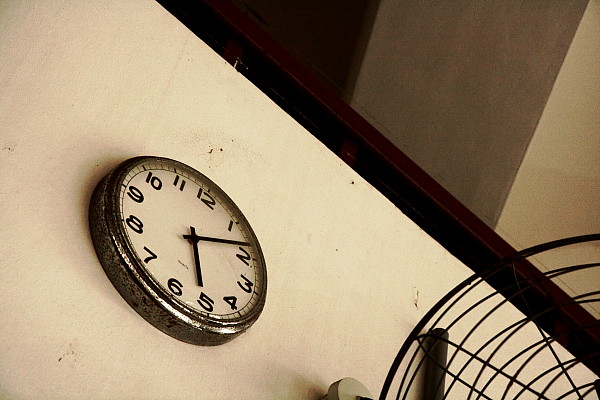The sepia-toned photograph captures an old, rusted wall clock with a metallic silver rim and a white face adorned with black hands and numbers, displaying the time as 5:08. The angle of the shot is from below, looking up, which lends a unique perspective. This clock, reminiscent of those found in old classrooms or office buildings, is mounted on a dirty, white wall that shows signs of age and neglect, evidenced by dirt specks and an overall grimy appearance. Adjacent to the clock is a partial view of a vintage metal fan, enclosed in a wire cage, adding to the antiquated ambiance. Above, a wooden beam runs across the top, enhancing the rustic aesthetic of the scene.